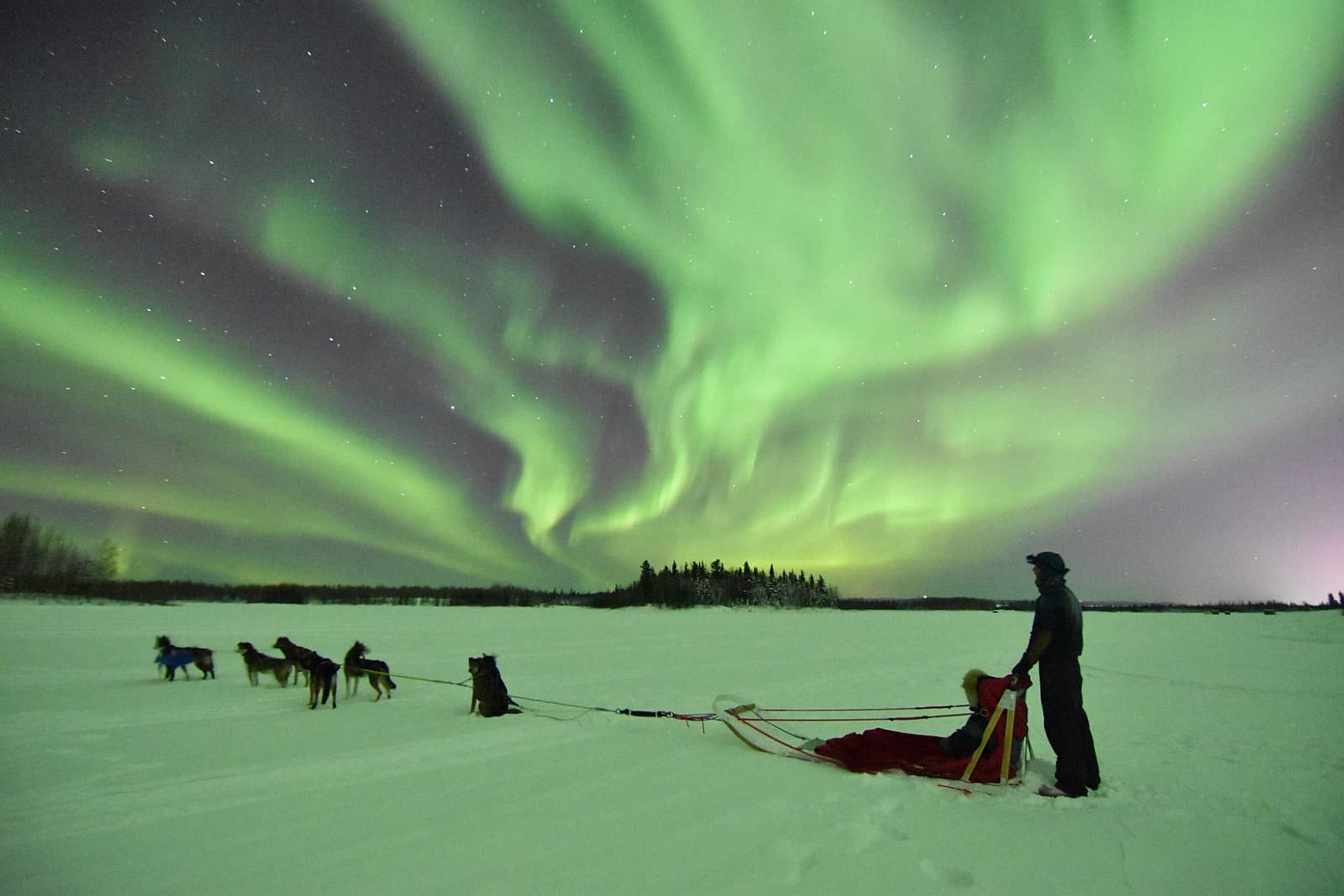The photograph captures an enchanting winter night scene in a snow-covered field, where a man dressed in protective winter gear stands at the back of a lightweight sled, tightly gripping the handle. This sled is pulled by a team of six husky dogs whose silhouettes appear dark against the snowy landscape. Seated comfortably inside the sled is another individual, wrapped in a red coat with a furry hood, possibly sitting on or wrapped in a red blanket. The sky above is a mesmerizing display of the aurora borealis, casting vivid green and yellow waves that fill the night sky and reflect onto the minty green snow below. The sky's non-aurora sections reveal deep shades of purple and black, dotted with countless twinkling stars. In the distance, a tree line and clumps of forest are faintly visible, including a distinct mound crowned with trees towards the horizon. Together, these elements combine to create a serene and captivating winter tableau.